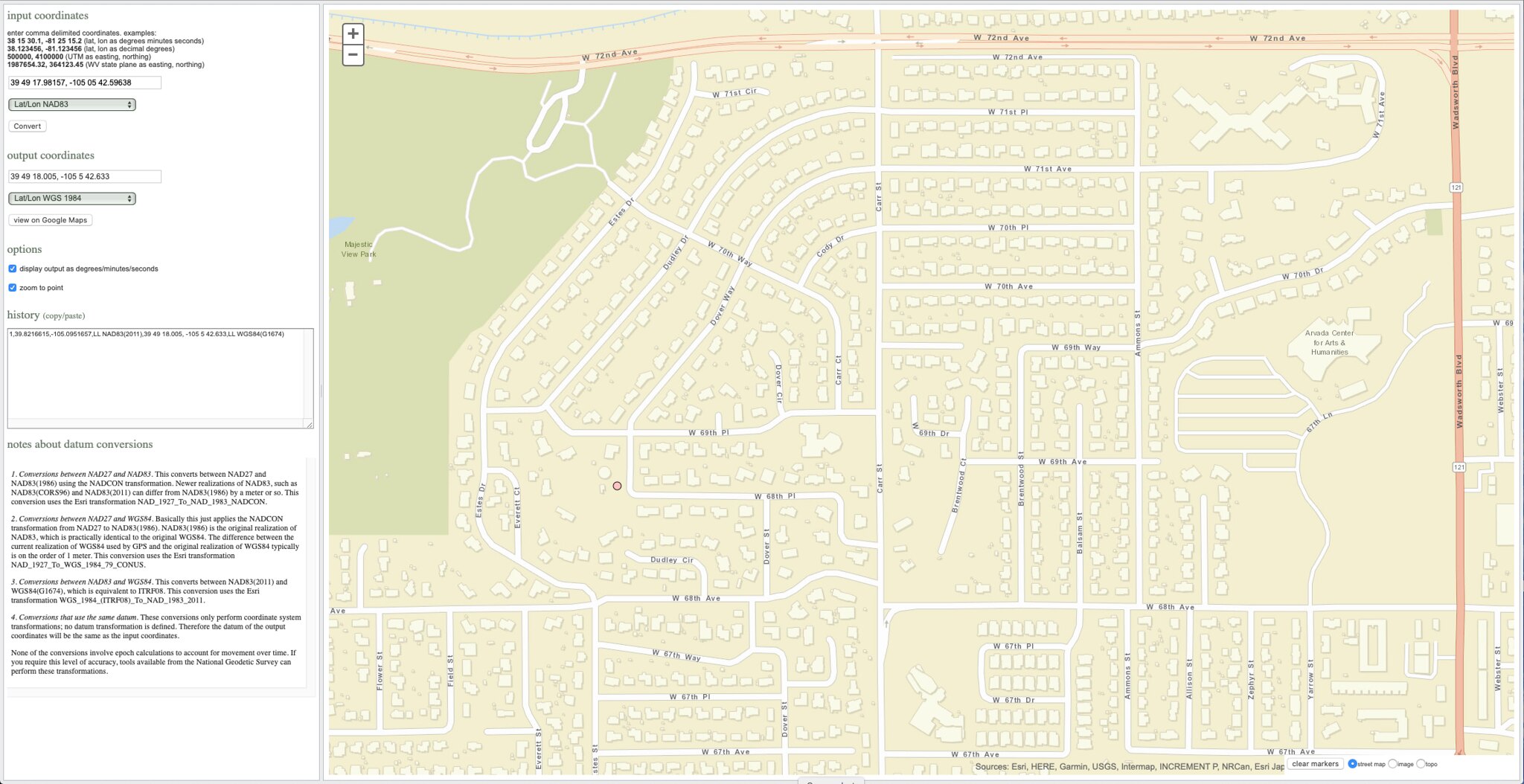This detailed screenshot of a complex map showcases an intricate web of information. At a glance, the map is densely packed with GPS coordinates and cryptic notes pertaining to various conversion factors used during its creation. In the bottom right corner, a barely legible key offers explanations and cites sources, including Garmin and USGS, although additional sources remain obscured. 

The map predominantly features a sprawling neighborhood, intersected by numerous streets and displaying a park situated in the upper left-hand quadrant. Notably, no distinct city names are included in this map. The rightmost eighth of the image is dedicated to detailed GPS coordinates and additional data regarding the conversion factors applied. Adjacent to these coordinates on the upper left side, two buttons allow for zooming in and out, providing greater control over the map’s view.

A single freeway runs vertically along the right edge of the map, serving as a significant landmark amidst the residential streets and green spaces. This detailed and layered map offers a blend of natural and urban elements, interspersed with technical details that cater to a specialized audience.